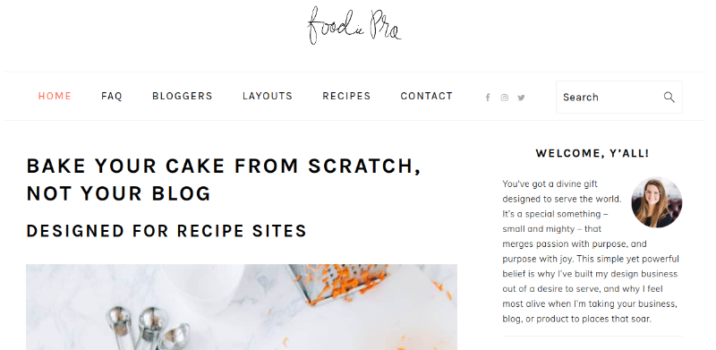Screenshot of a website with a clean, white background and various elements designed for food enthusiasts. The website header features the "Foodie Pro" logo and navigation links in black including "Home," "About," "FAQ," "Bloggers," "Layouts," "Recipes," and "Contact." Social media icons for Facebook, Snapchat, and Twitter are also displayed. A search bar with a magnifying glass icon is positioned prominently.

The main header reads, "Bake Your Cake from Scratch, Not Your Blog," indicating the site is tailored for recipe bloggers. Below, an image of a grater with freshly grated carrots adds a touch of culinary activity.

The welcome message states: "Welcome y'all! You've got a divine gift designed to serve the world. It's a special something small and mighty that merges passion with purpose and purpose with joy. This simple yet powerful belief is why I've built my design business out of a desire to serve and why I feel most alive when I'm taking your business, blog, or product to places that soar."

On the side, there is a profile picture of a smiling woman with long blonde hair, proudly displaying her teeth. She is the likely owner and creator of the site.